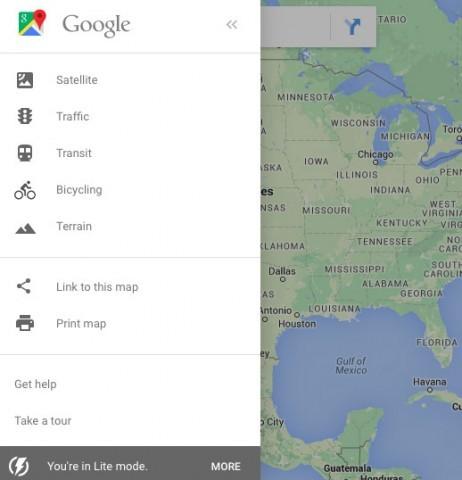**Caption:**

This detailed screenshot from Google Maps captures a view predominantly focused on the Midwest of the United States. The image, which is slightly taller than it is wide, is structured into two main sections: a side panel on the left and a map on the right.

The side panel occupies approximately 55% of the image and has a white background, segmented into five distinct sections by light gray lines extending horizontally. The bottom section of the panel is set apart with a dark gray background and white text. In the lower left corner of this section, a lightning bolt icon within a circle is accompanied by the text "You're in LITE mode." On the right, it reads "MORE" in all caps.

The top section showcases the Google Maps icon, a small multicolored square with a red pin, and the word "Google" in its recognizable corporate font. To the far right of this section, there are two arrowheads pointing to the left.

Below this, the second section lists five icons with corresponding labels: 
- Satellite (represented by a dark gray square with a white mountain and rays)
- Traffic (a traffic light icon)
- Transit (a front view of a bus or subway)
- Bicycling (a side view of a person on a bicycle)
- Terrain (overlapping mountain icons).

The third section features two rows, with the labels "Link to this map" and "Print map," each tagged with unique icons (a triangular shape made of connected dots for linking and a printer for printing). The fourth section includes two options, "Get help" and "Take a tour," aligned with the icons above but without any symbols.

Covering about 45% of the image, the map itself is color-coded, showing a broad area from the tip of Florida to Canada, and from parts of Nebraska, Kansas, Oklahoma, and Texas to the Gulf of Mexico. The map extends to parts of Central America, including Guatemala and Honduras, and features Cuba near the lower right corner. Key cities like Houston, Dallas, and Chicago are marked, while state names appear in all caps. The land is shaded in various greens and some yellowish tones towards the Midwest, with water bodies like the Great Lakes and the Gulf of Mexico visible and labeled. No roads are displayed, ensuring a clean, geographical focus.